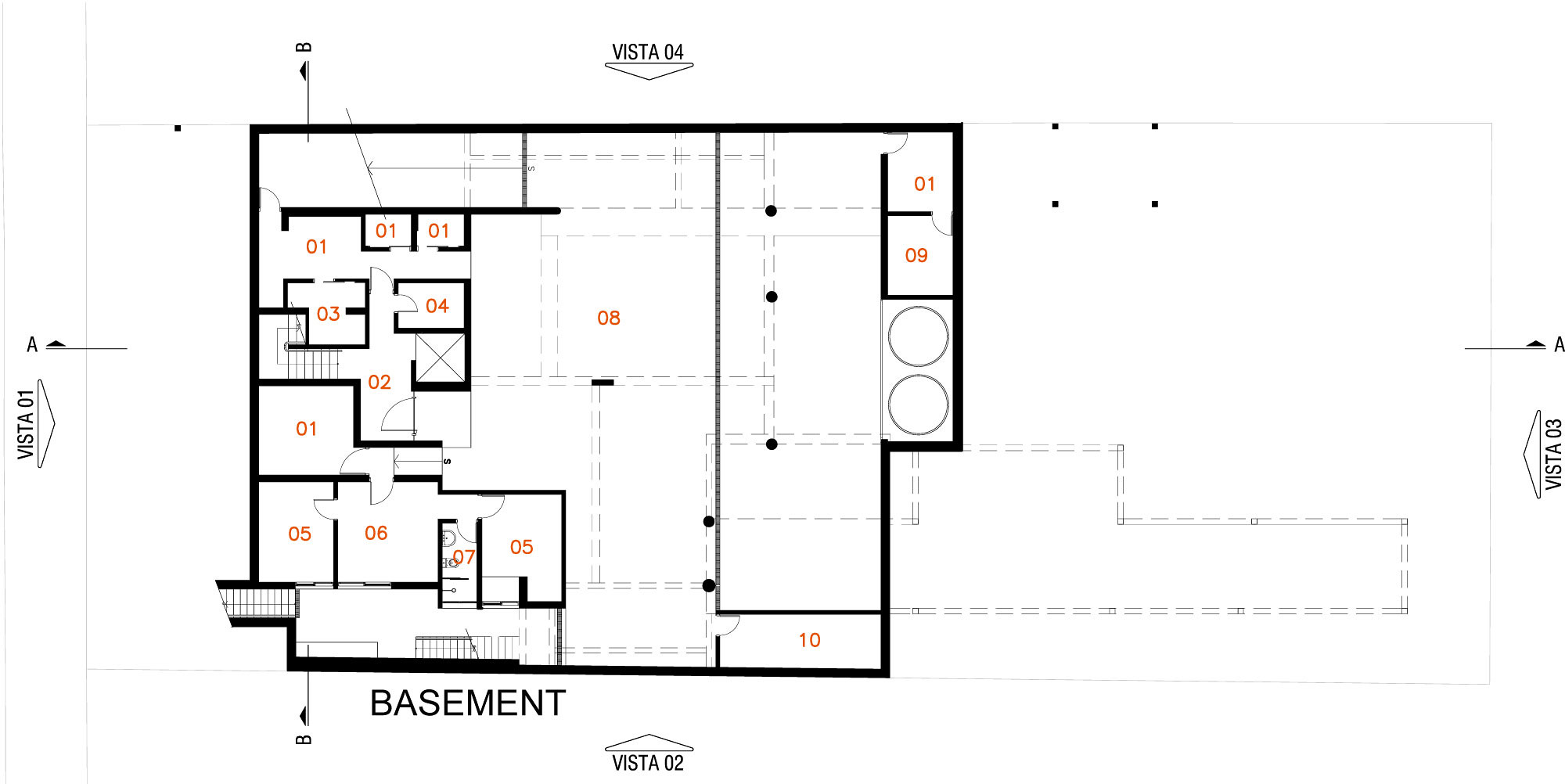This image displays a detailed blueprint-style layout of a home, depicted on a clean white background. The home's floor plan is outlined in black, with multiple annotated points for clarity.

On the left side of the image, a label "Vista 01" with the letter "A" points to an open area outside the home, suggesting a view or scenic spot. At the bottom of the blueprint, label "B" directs attention to the "basement," which is connected by a flight of stairs. Adjacent to the basement, there is an arrow labeled "Vista 02" indicating another view within the property.

Beside the basement area, the plan shows a series of doors leading to four rooms labeled "05," "06," "07," and another "05." Rooms "05" and "07" are solely accessible via the basement. Room "06" connects to another room marked "01," which opens up to a primary area designated as "08."

From the main area "08," there are access points leading left to Room "02" and a staircase descending to Room "03." Additionally, "08" connects upward to three rooms labeled "01," with one leading to Room "04." The top of the home contains an exit marked by "Vista 04," with an arrow indicating a downward view.

On the right side of the blueprint, an expansive open area, possibly a yard, is marked "Vista 03" with another "A" pointing towards it. From the primary room "08," Room "10" can be accessed directly at the bottom right corner.

Moreover, there is a partitioned section with Room "01" connecting to Room "09," suggesting a distinct but interconnected area within the home.

Overall, the blueprint provides a comprehensive overview of the home's layout, including detailed room connections and various scenic viewpoints labeled as 'Vistas.'